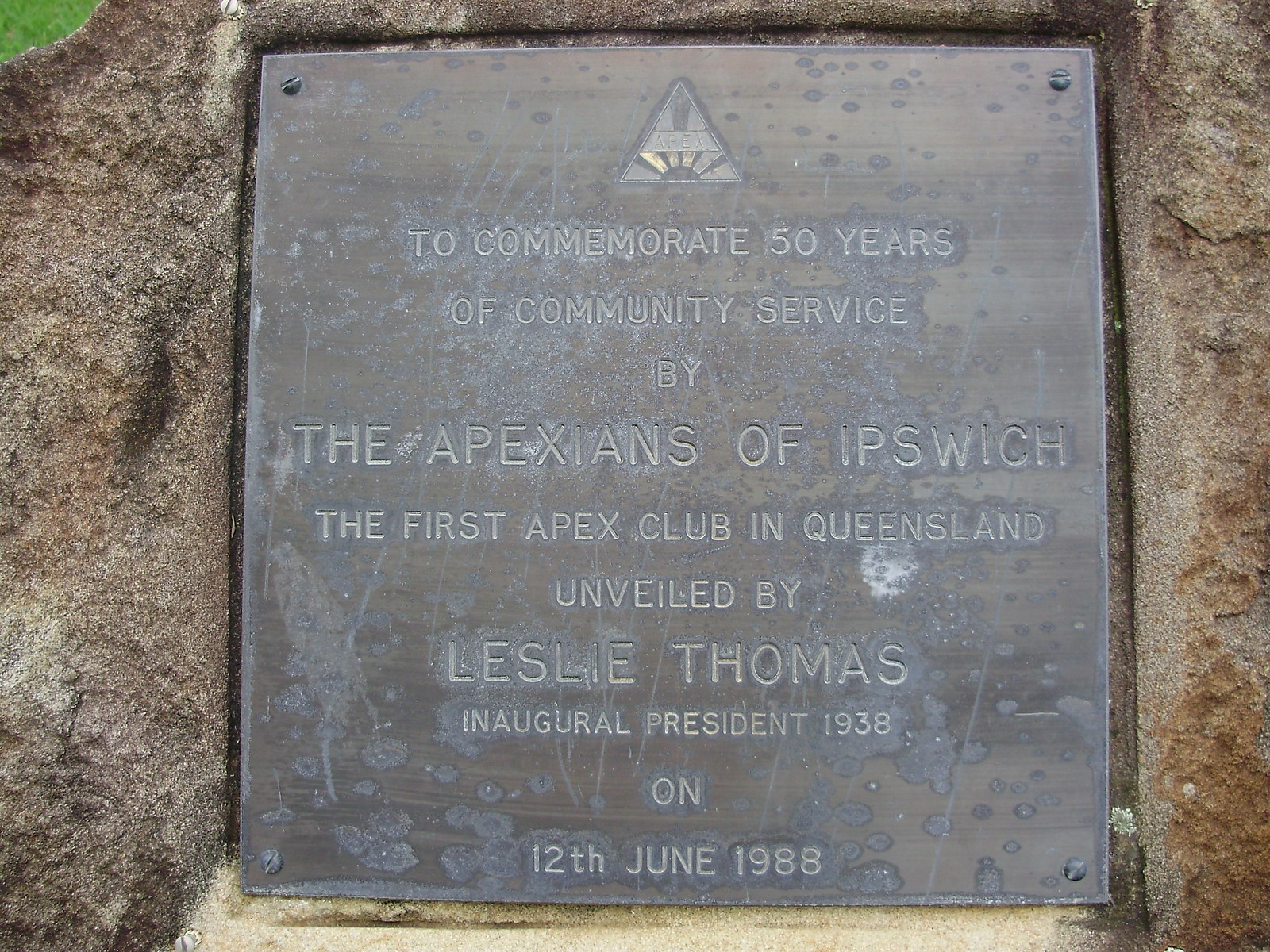This photograph depicts a worn, engraved black stone plaque set against a brown stone wall with some green vegetation visible in the upper left corner. The plaque, which appears to be quite aged, is adorned with white and water spots. It features an inscription commemorating 50 years of community service by the Apexians of Ipswich, the first Apex club in Queensland. The dedication was unveiled by Leslie Thomas, the inaugural president, on June 12, 1988. The top of the plaque is marked with a small triangle, and it is well-embedded within the wall, suggesting it may have been installed in a hollowed-out section of the stone.